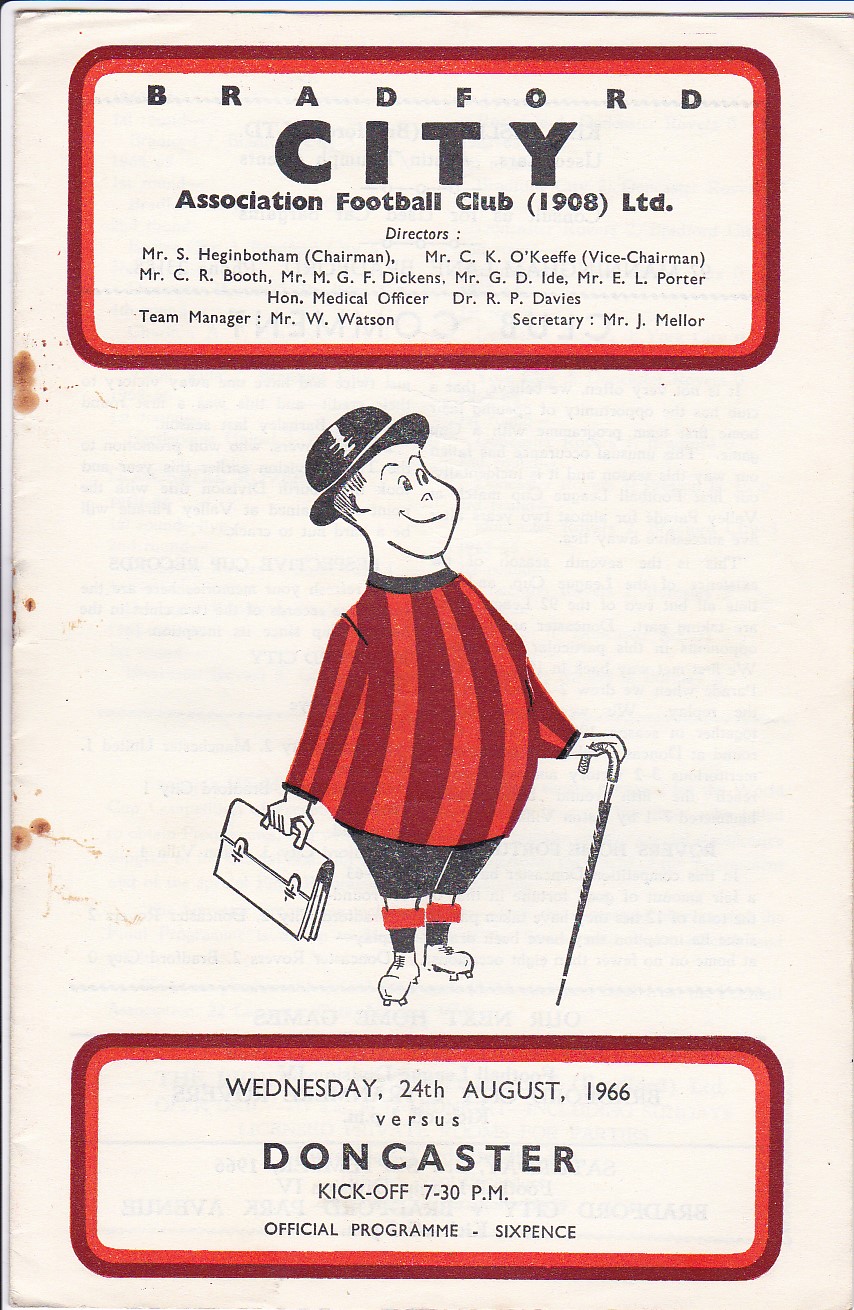This image is a scanned cover of an old football program for the Bradford City Association Football Club. The cover, which is printed on off-white paper now aged and somewhat faded, features black text with red outlined trim boxes at the top and bottom. At the top, it prominently displays "Bradford City Association Football Club 1908 Limited." Below this, a series of director names are listed: Mr. S. Heitenbaum (Chairman), Mr. C.K. O'Keefe (Vice Chairman), Mr. C.R. Booth, Mr. M.G.F. Dickens, Mr. G.D. Iden, Mr. E.L. Porter, with Dr. R.P. Davies as the Honorable Medical Officer, Mr. W. Watson as the Team Manager, and Mr. J. Miller as the Secretary. 

The central portion of the cover features a classic, vintage cartoon drawing of a man dressed in a red and white striped jersey, black shorts, and red socks, accessorized with a black bowler hat, a briefcase in one hand, and an umbrella in the other, held like a cane. The character is facing away from the viewer, looking to the right. 

At the bottom of the cover, the details of the event are given: "Wednesday, 24th August 1966 vs Doncaster," with a kickoff time of 7:30 PM. The price of the official program is listed as sixpence. Notably, there is evidence of rust from old staples, marking where the pages were once bound together.